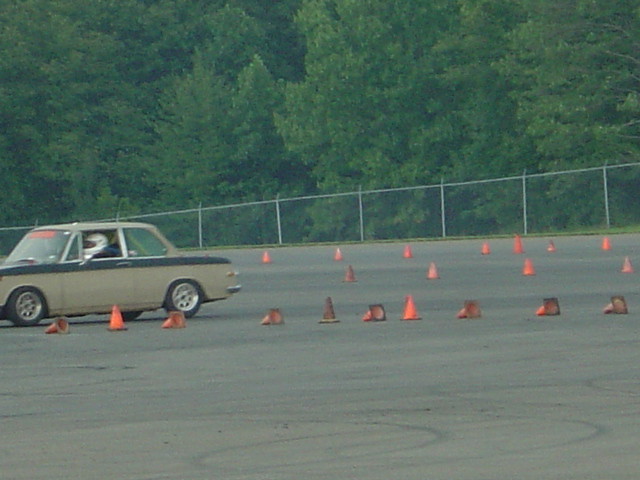The photograph captures an old, gray and tan two-door mini sedan driving through a makeshift obstacle course in an empty parking lot. The driver, who is wearing a white helmet, is navigating around roughly 25 orange cones dispersed throughout the lot, with many of the cones laying knocked over. The background is filled with a dense forest of large, green trees and a chain-link fence running parallel to the scene. The car, which has large wide windows, also features a red sticker or sign on the top of the front dashboard, adding a touch of color to the otherwise muted vehicle.